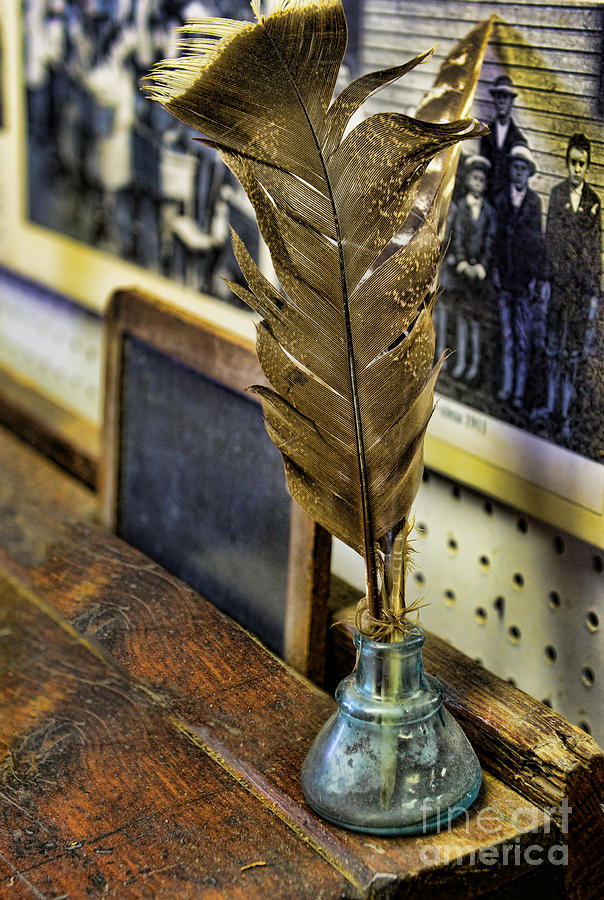The image appears to depict a historically themed scene set on an old, worn table or desk, likely situated in a museum or similar setting. Prominently featured in the foreground is an empty ink well containing quills adorned with thick brown and white feathers. The desk is rustic and aged, complemented by an equally old chair. Behind the desk, there is a pegboard, possibly with holes for hanging items, and a small chalkboard-like object. An aged, black-and-white photograph hangs on the wall, displaying a family portrait that includes several children and a man, all dressed in period-appropriate attire, with three of the boys wearing hats. The photo is partially out of focus, enhancing the nostalgic and historical ambiance of the scene. The bottom of the image features the text "Fine Art America," adding to its artistic and antiquarian appeal.